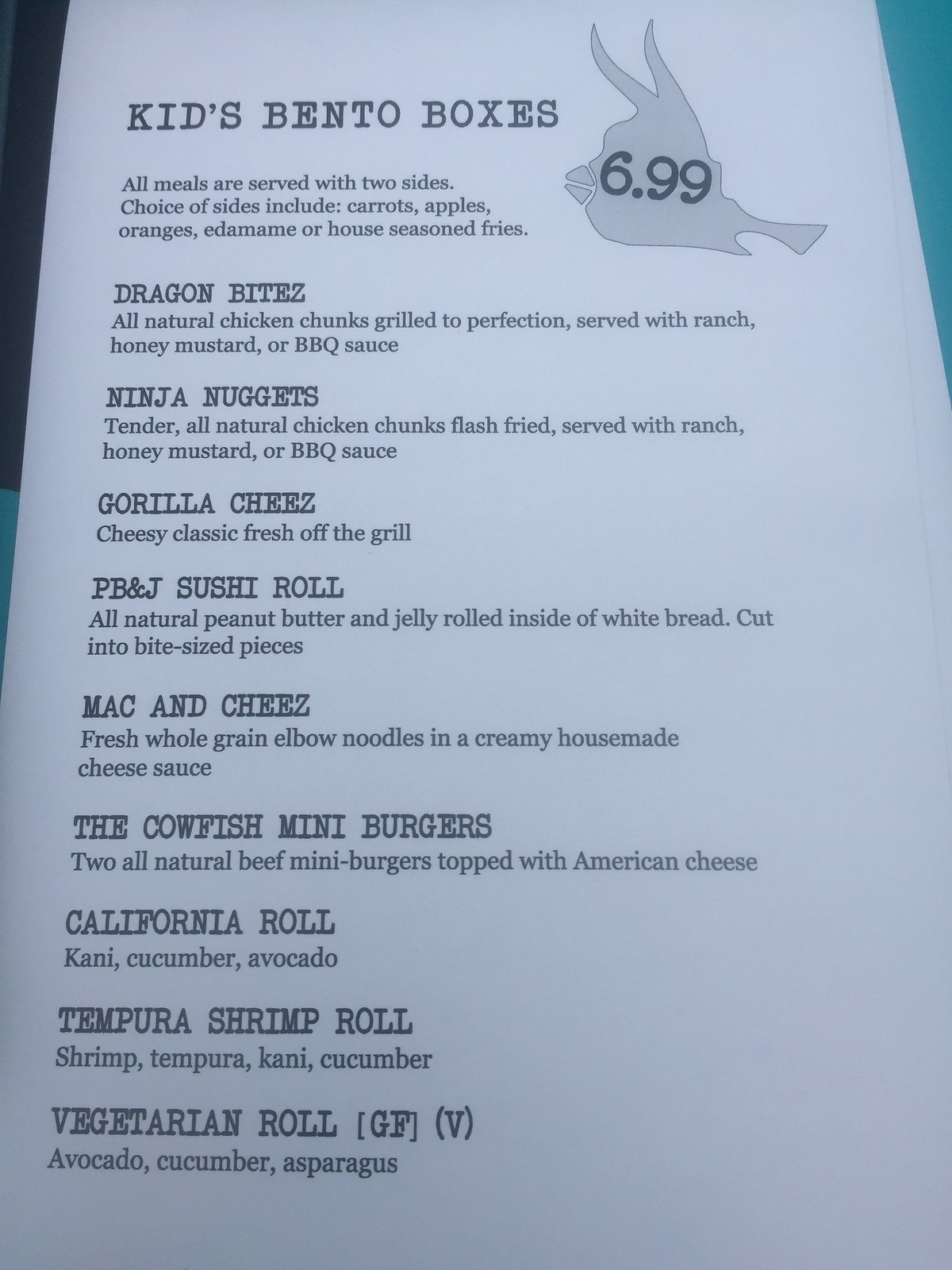This photograph showcases a restaurant menu designed specifically for kids, with the heading "Kids Bento Boxes $6.99" prominently displayed at the top. Each meal option is accompanied by a choice of two sides, including carrots, apples, oranges, edamame, or house-seasoned fries.

The menu features the following bento box choices:

1. **Dragon Bites**: All-natural chicken chunks, grilled to perfection and served with a choice of ranch, honey mustard, or BBQ sauce.
2. **Ninja Nuggets**: Tender, all-natural chicken nuggets, flash-fried and served with a choice of ranch, honey mustard, or BBQ sauce.
3. **Gorilla Cheese**: A cheesy classic, fresh off the grill.
4. **PB&J Sushi Roll**: All-natural peanut butter and jelly, rolled inside white bread and cut into bite-sized pieces.
5. **Mac and Cheese**: Fresh, whole-grown elbow noodles in a creamy house-made cheese sauce.
6. **The Cowfish Mini Burgers**: Two all-natural beef mini burgers topped with American cheese.
7. **California Rolled**: Cani, cucumber, and avocado.
8. **Tempura Shrimp Roll**: Shrimp tempura, cani, and cucumber.
9. **Vegetarian Roll (GF, V)**: Avocado, cucumber, and asparagus.

The menu is printed on off-white paper with a slight blue tint, and all text is rendered in black ink.